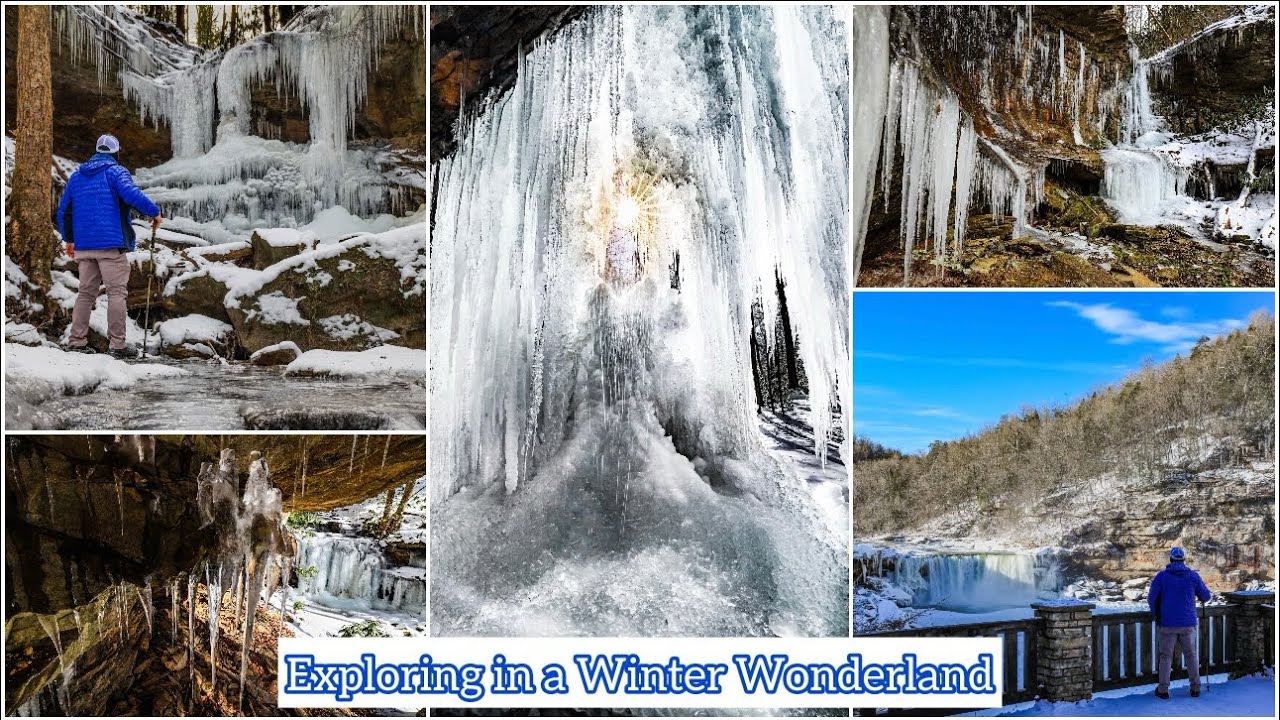This collage, titled "Exploring in a Winter Wonderland" in blue outlined letters on a white background, features a series of wintery images filled with snow and ice. The top left image showcases a man wearing a blue ski jacket, tan pants, and a baseball cap, holding a hiking stick. He stands beside a brown tree trunk with icicles dangling overhead, looking over a snowy stream. The center and largest image reveals the inside of a cave, dominated by a large sheet of icicles with sunlight filtering through. To its right, the top picture captures the interior of a cave or a cliff's edge, characterized by dark brown stone and numerous icicles. Below, on the far right, the same man in his blue jacket and tan pants stands on a deck with brick columns and a wooden fence, gazing at a waterfall that cascades into white foam or may be frozen. Behind him, a sparsely vegetated hill rises against a clear blue sky with streaks of white clouds. The bottom image in the center portrays icicles from within a cave-like structure, emphasizing the intricate frozen details.